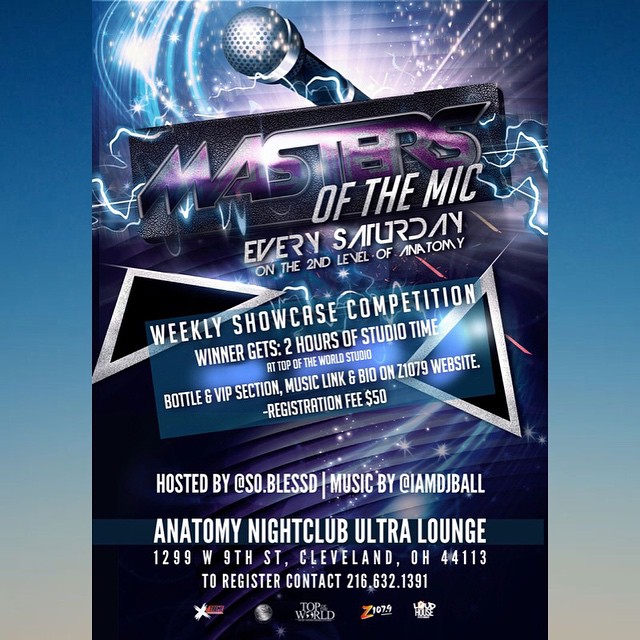This square-shaped flyer, measuring approximately five inches by five inches, advertises an event called "Masters of the Mic" held at Anatomy Nightclub Ultra Lounge, located at 1299 West 9th Street, Cleveland, Ohio 44113. The background transitions from dark blue at the top, lightening to light blue in the middle, and finally to light gray at the bottom. At the top center of the flyer, a bold, textured heading reads "Masters of the Mic," with energy trails and sparks radiating from the text. Just above this, a microphone graphic extends from a black rectangle labeled "masters" in purple text.

Below the main title, the flyer announces that the event takes place every Saturday on the second level of Anatomy. It features a weekly showcase competition, with the winner receiving two hours of studio time at Top of the World Studio, a bottle and VIP section, as well as a music link and bio on the Z107.9 website. The registration fee for the event is $50.

Additional information highlights that the event is hosted by @so.blessed and music is provided by @imdjball. The flyer provides a registration contact number: 216.632.1391. At the bottom of the flyer, sponsor logos are displayed, including those for Extreme, a silver globe, Top of the World, Z107.9, and Loud House.

This vibrant and dynamic flyer successfully conveys the details of the lively event through energetic graphics and well-organized text.